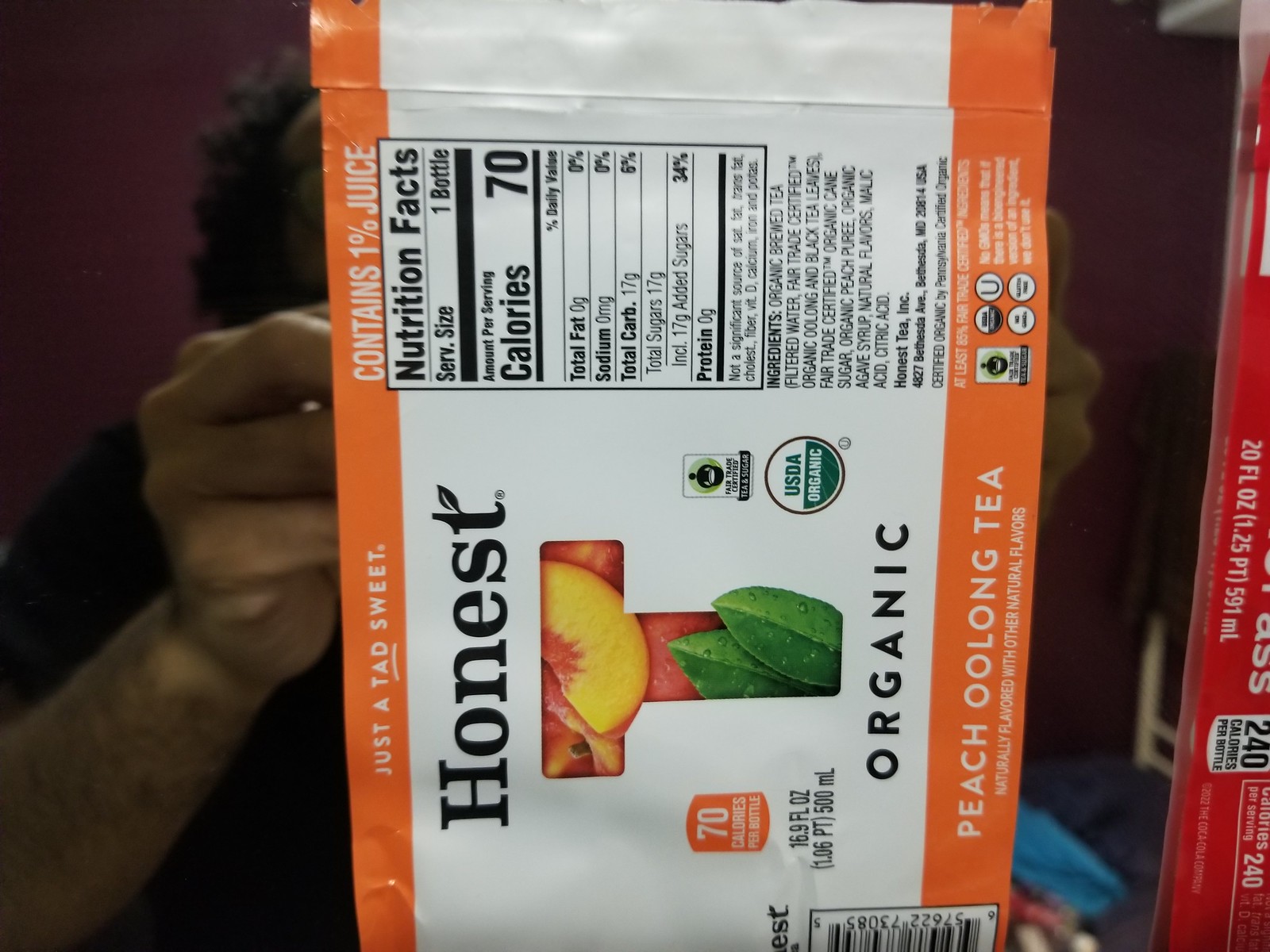In this image, a case of Honest Organic Iced Peach Oolong Tea is held upright but turned sideways, necessitating a head tilt to the left to read the labels properly. The case is grasped from behind by a hand, where we can see the top side of a couple of fingers and part of the forearm extending from the bottom left corner. The top right section of the image shows a partial view of outer hair strands and a black t-shirt, with the case obscuring the person’s face. The case features orange stripes along the left and right edges and a predominantly white background. In black text, it states "Honest" with the 'T' stylized with different fruits. Below, it reads "Organic" followed by "Peach Oolong Tea," with "Oolong" spelled without the initial 'C' as "O-O-L-O-N-G." On the right side of the case, the nutrition facts label is visible, topped with a note that says "Contains 1% juice." The extreme right edge of the image reveals a hint of another red container.